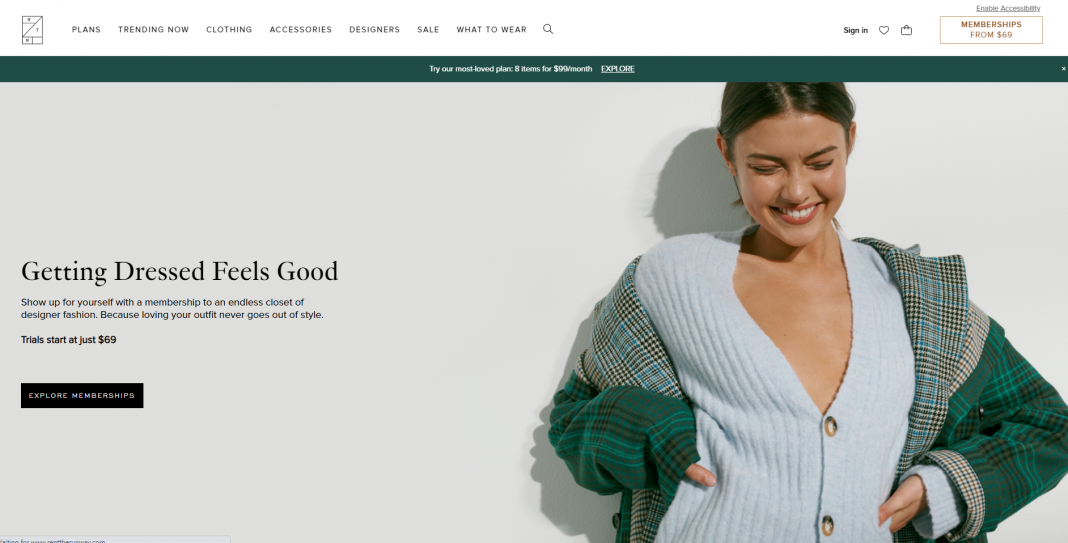**Screenshot of a Fashion Website**

The screenshot captures a vibrant and sophisticated fashion website. At the top left corner, a rectangular logo marks the page, though the company's name is not visible. The main navigation bar spans the top of the page, featuring categories in the following order from left to right: Plans, Trending Now, Clothing, Accessories, Designers, Sale, What to Wear, and a search icon. Adjacent to these, user options include sign-in, a heart icon for a wishlist, and a suitcase or bag icon representing the shopping cart. A notable detail on the far right is the membership offer, starting at $69.

Beneath the navigation bar, a prominent banner ad invites users to try their most loved plan, offering eight items for $99 per month, accompanied by an "Explore" button.

The main feature image below showcases a smiling young woman bathed in sunlight, donning a button-up sweater with a low neckline, layered elegantly with a plaid jacket. She stands against the clean simplicity of a white background.

To her right, the viewer is engaged by the text stating, "Getting dressed feels good. Show up for yourself with a membership to an endless closet of designer fashion because loving your outfit never goes out of style. Trials start at just $69." A black "Explore Memberships" button is conveniently placed under this text, encouraging further interaction.